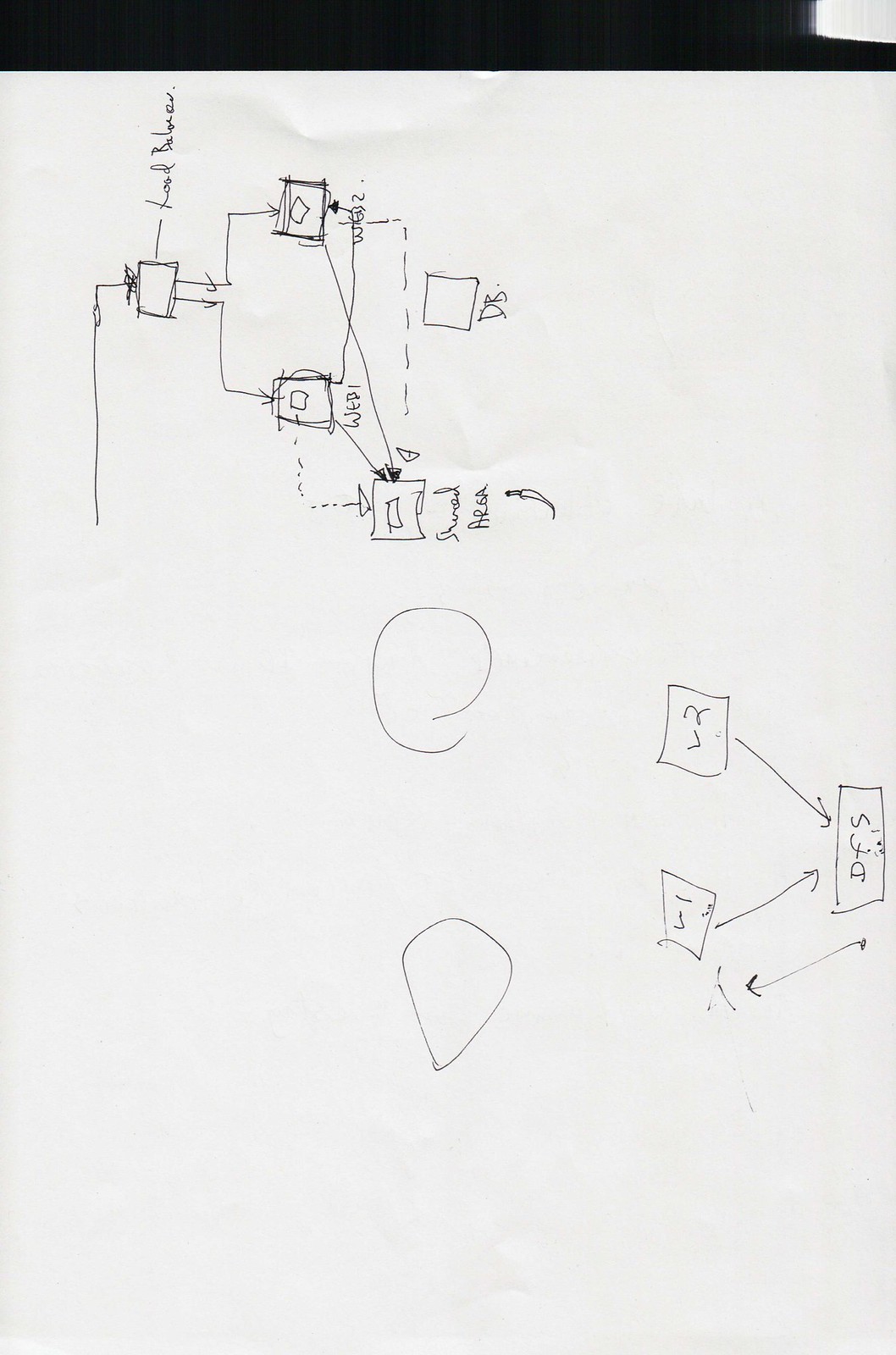This photograph captures a piece of white unlined paper filled with roughly drawn diagrams, rotated 90 degrees. The diagrams, all rendered in black ink, feature various interconnected geometric shapes, predominantly squares, connected by solid and dashed lines. In one corner, there is a single prominently drawn circle. At the top right of the sheet, the words "load balance" are written in black script with a short horizontal line leading to a square. The upper portion of the image reveals a dark or black background that could be a tabletop, accented by a small white rectangular section positioned at the top right. The overall depiction is monochromatic, emphasizing the stark contrast between the black ink and the white paper.